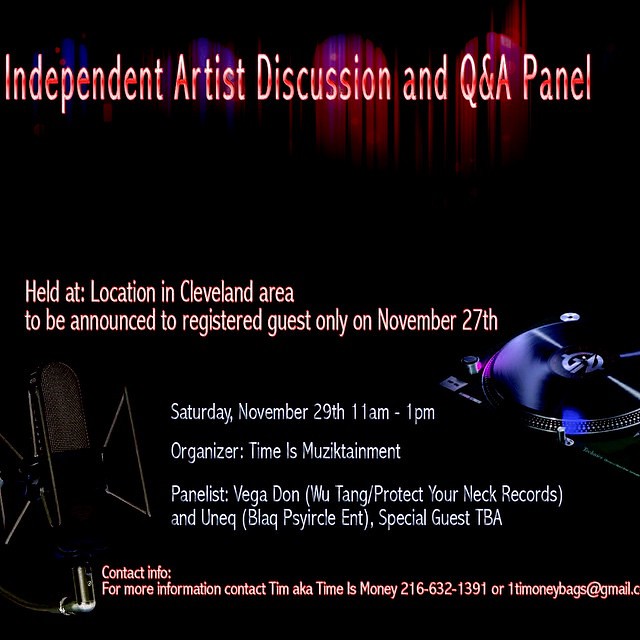The image is a dark, modern flyer with a black background featuring prominent text in light pink, red, and white. At the top, bold letters announce, "Independent Artist Discussion and Q&A Panel," accentuated by vertical streaks of color. The event details are described in white text: it will take place in the Cleveland area, with the exact location revealed to registered guests only, on November 27th. Further down, the flyer specifies the event date as Saturday, November 29th, from 11 a.m. to 1 p.m. representing a discrepancy in dates which should be verified. 

An illustration of a turntable with a record is located to the right, accompanied by images of a microphone in the lower left corner, adding a musical theme. The panelists include names like Vega, Don (affiliated with Wu-Tang Project and Protect Your Neck Records), and UNEC (from Black Psy Circle Entertainment), with a special guest to be announced. Organizing is handled by Musictainment. The contact info at the bottom provides details to reach Tim, also known as Time is Money, with a phone number and email in red, maintaining the flyer’s color scheme.